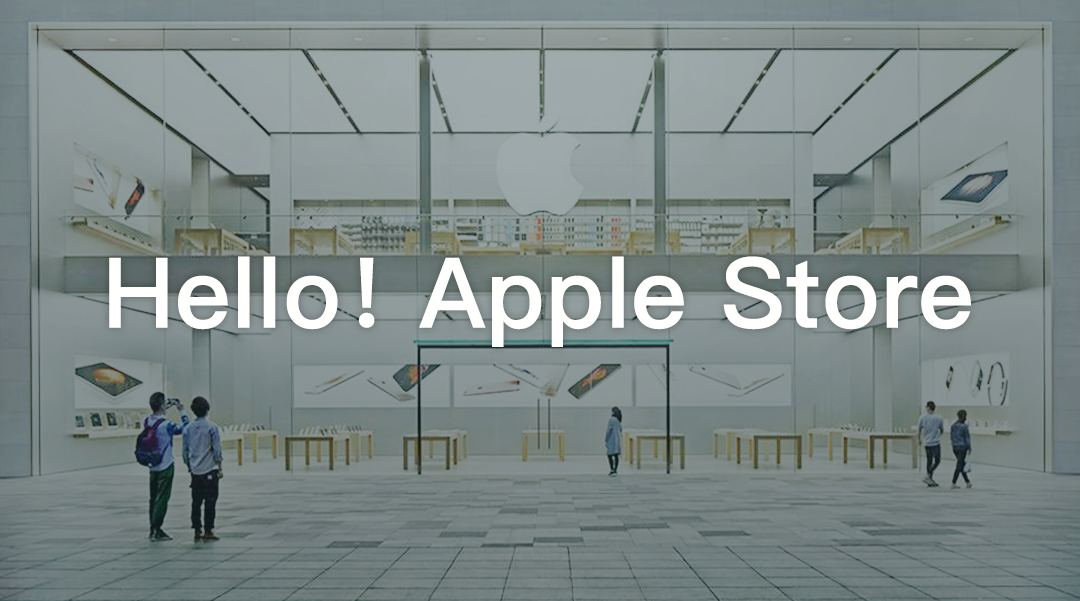The image captures a two-level Apple Store, characterized by its iconic Apple logo prominently displayed on the large glass facade. The front of the store is entirely made of glass windows, allowing a clear view into the interior. Inside, large posters display various Apple phones and accessories. The store is meticulously organized with several wooden tables, presumably showcasing an array of Apple products such as phones and tablets for customers to try out.

In the foreground, outside the store, two men are visible. One man, who has a backpack and a camera in his hand, stands gazing up at the store. To the left, a woman in a blue coat is positioned just at the entrance, peering into the store. To the right, a man and a woman, who are wearing blue shirts with varying shades, walk past the store. The man in the lighter blue shirt glances back over his shoulder, looking into the store as they move along.

The interior of the store appears to be pristine and well-organized. It is devoid of customers, presenting an austere yet inviting atmosphere, with large posters adorning the walls and wooden tables neatly arranged to exhibit Apple's latest technology.